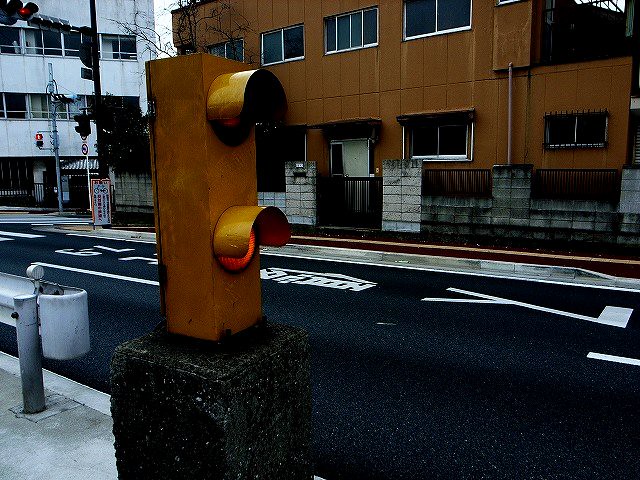In the photograph, a bustling street scene is depicted, likely outside of the United States given the unique traffic features. The street at the bottom is surfaced with blacktop and prominently marked with clear white lines, which include partially visible numbering, possibly "79" on the left-hand side. Dominating the foreground is a distinctive traffic light mounted on a low-standing, dark yellow, concrete structure. This traffic light, standing just slightly taller than an average person, features only two lights, with the lower red light currently illuminated despite the absence of any vehicles in the frame.

Across the street, a guardrail is visible, providing a boundary just behind the traffic light. Beyond the guardrail stands a medium brown building characterized by a fenced-in patio area. The patio is enclosed with black railings and supported by robust concrete posts. The overall scene captures the intricacies of the urban environment, hinting at a non-American setting through its distinct infrastructural elements.